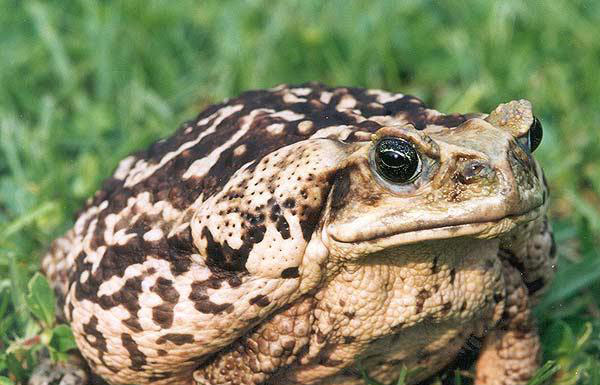The photograph captures a grumpy-looking toad with a wide mouth and a stout, green body set against a backdrop of blurred grass. The toad, which sports a scaly appearance, has a brown back adorned with clear spots. Its big, black eyes with protective membranes and prominent nostrils add to its expressive demeanor as it looks off towards the right. The scene evokes a sense of the creature simply relaxing in a grassy field, perhaps contemplating its next move.